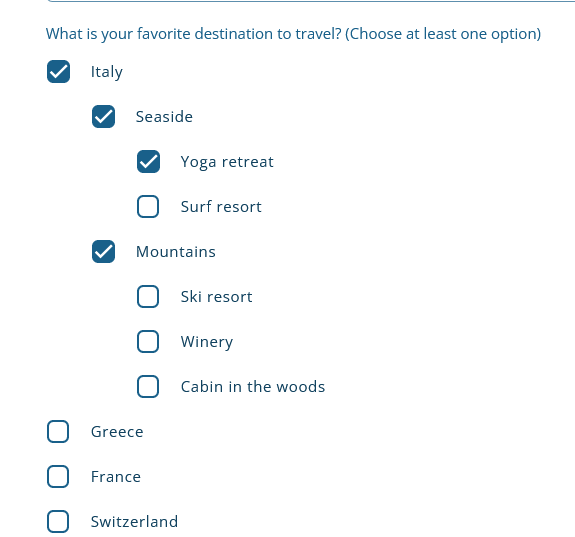The image displays a screen with a travel survey question, asking "What is your favorite destination to travel?" There is a bracketed instruction to "choose at least one option."

Below the question is a hierarchical list of travel destinations with corresponding checkmarks indicating selections. The structure is as follows:

1. **Italy** (selected with a blue tick)
   - **Seaside** (selected with a blue tick)
     - **Yoga Retreat** (selected with a blue tick)
     - **Surf Resort** (not selected)
     - **Mountains** (selected with a blue tick)
       - **Ski Resort** (not selected)
       - **Winery** (not selected)
       - **Cabin in the Woods** (not selected)
2. **Greece** (not selected)
3. **France** (not selected)
4. **Switzerland** (not selected)